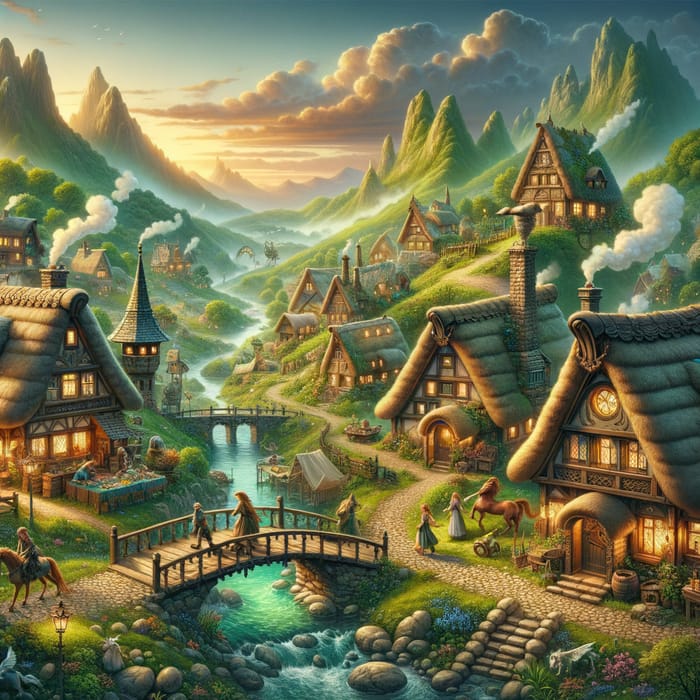The detailed image depicts a picturesque medieval Scandinavian village nestled along the sloping green sides of mountainous hills. The village features two to three-storied cottages, with steep thatched roofs adorned with ornamental strips of wood resembling the prows of Viking longboats. These charming homes are tiered along both sides of a narrow, blue-green stream that flows through the center of the scene, accented by little rocks. Two stone-paved bridges cross the stream, one in the foreground bustling with people walking and riding horses. Smokestacks protrude from the cottages, emitting plumes of white smoke into the crisp air. The sky above transitions from a yellow hue on the left to a deep blue on the right, interspersed with clouds that shift from orange-yellow to gray. The overall composition, possibly a painting or video game frame, blends natural beauty with the quaint architectural charm of a historical village.